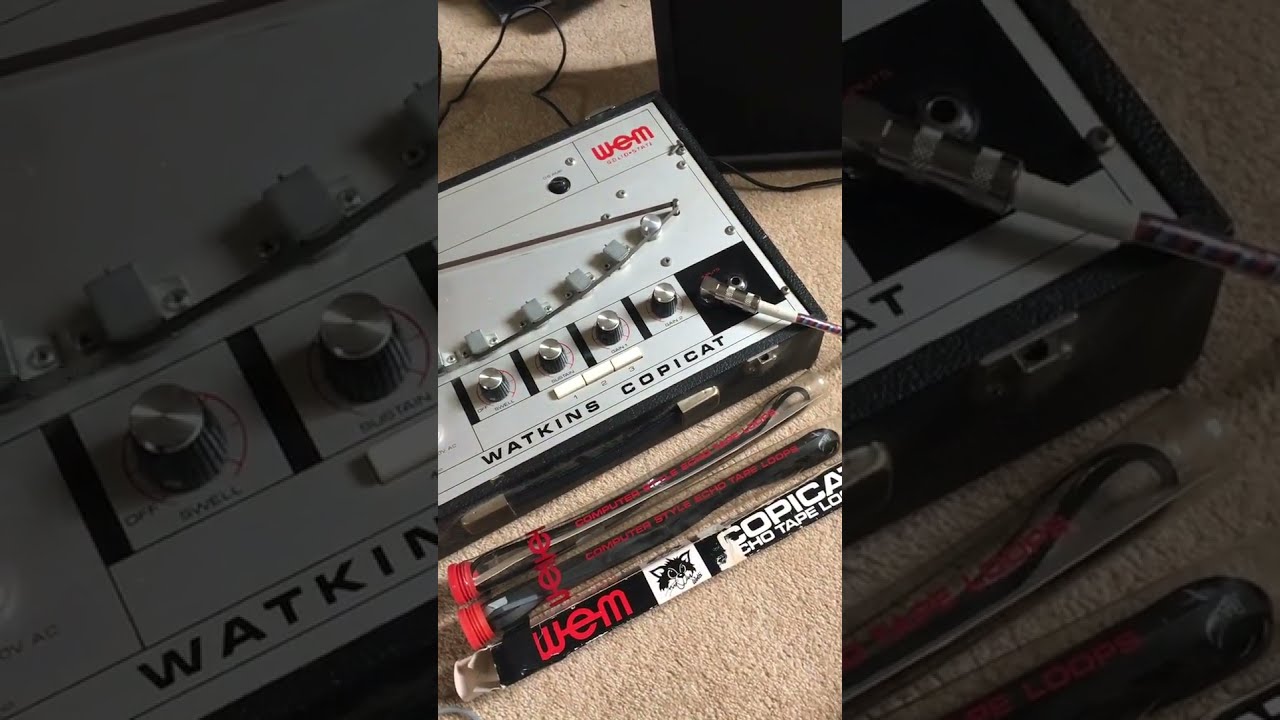The image showcases a close-up view of vintage musical equipment placed on a beige carpet. Central to the composition is a piece of stereo equipment labeled "Watkins Copicat." The device features a brushed silver top with four black-and-silver knobs and three white buttons labeled 1, 2, and 3. Encased in a black leather holder resembling a briefcase with a handle on the side, the equipment appears portable, capable of being closed and locked for easy transport. Also notable is an unplugged cable lying next to an input port on the device.

Below the main equipment, three clear plastic tubes with red caps, containing black tape loops, are arranged diagonally. The tubes are inscribed with "W.E.M." in red text. Additionally, a partially visible box marked "W.E.M. Copycat" with a logo of a cat and the words "ECHO TAPE" lies nearby. The setting appears well-lit, likely from natural or artificial light, enhancing the visibility of the detailed features of the equipment and tubes.